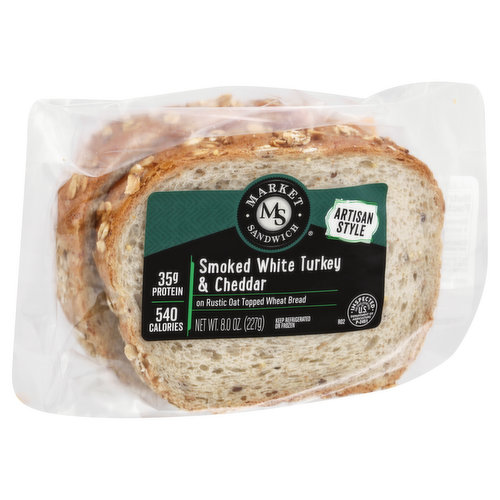This photograph showcases a pre-packaged, single-serve sandwich enclosed in clear, airtight packaging, prominently displaying its fresh and appetizing appearance. The sandwich features a rustic oat-topped wheat bread, with visible oat flakes enhancing its artisanal appeal. The label, primarily in dark green and black, reads "Market Sandwich Artisan Style Smoked White Turkey and Cheddar on Rustic Oat Topped Wheat Bread." Nutritional details are highlighted on the label, specifying that the sandwich contains 35 grams of protein and 540 calories. The label further provides a net weight of 8.0 ounces (227 grams) and advises keeping the sandwich refrigerated or frozen. Quality assurance is noted with a USDA inspection. While the image does not reveal the sandwich's interior, the exterior bread appears hearty and delicious.